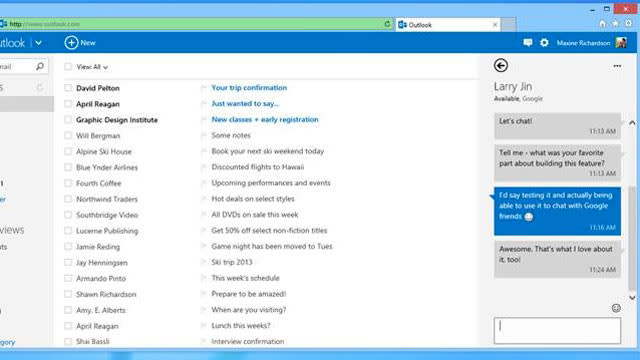Screenshot depicting an email client with a blue frame and navy blue header, resembling Microsoft Outlook. The interface is partially obscured with a left sidebar cutoff and a visible right sidebar highlighting a contact named Larry Jin. 

In the right sidebar, a chat window is open, featuring the following conversation:
1. Larry Jin: "Let's Chat" (11:13 AM).
2. Larry Jin: "Tell me what was your favorite part about building this feature?" (11:13 AM).
3. User Response (in blue): "I'd say testing it and actually being able to use it to chat with Google friends 😊" (11:16 AM).
4. Larry Jin: "Awesome. That is what I love about it too really!" (11:24 AM).

Below the conversation is a chat box for typing responses. 

The main content area, with a white background, displays an email list organized into two columns. Each row features a checkbox to the left of the sender's name and the subject line in blue text to the right:
1. David Pelton: "Your Trip Confirmation."
2. April Reagan: "Just Wanted to Say."
3. Graphic Design Institute: "New Classes + Early Registration."